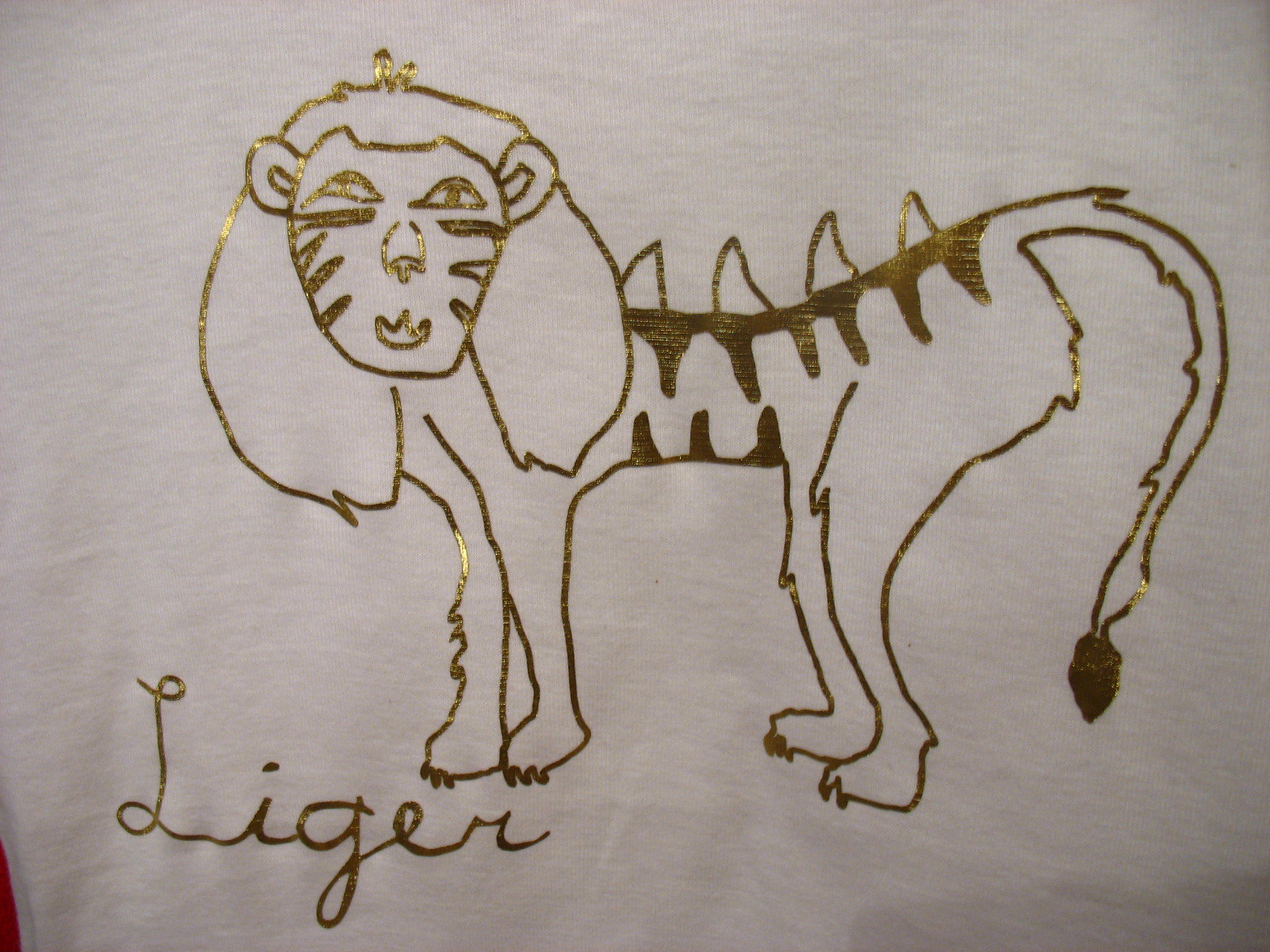The image features a horizontally aligned rectangular illustration on a white fabric, possibly a t-shirt. Depicted in gold-colored glitter paint or pen, is a comical cartoon character labeled "Liger" in cursive in the lower left-hand corner. The liger, a whimsical hybrid of a lion and a tiger, sports a voluminous mane framing its face, with tiger stripes adorning both its face and sides. The creature's body is tall and skinny, adorned with four bony protrusions or spikes along its back, resembling dorsal fins. Its long tail has a shaded tip, completing the fanciful design. The Liger faces the viewer with a partially side-turned body to the left, its playful and imaginative details rendered in glittery gold.